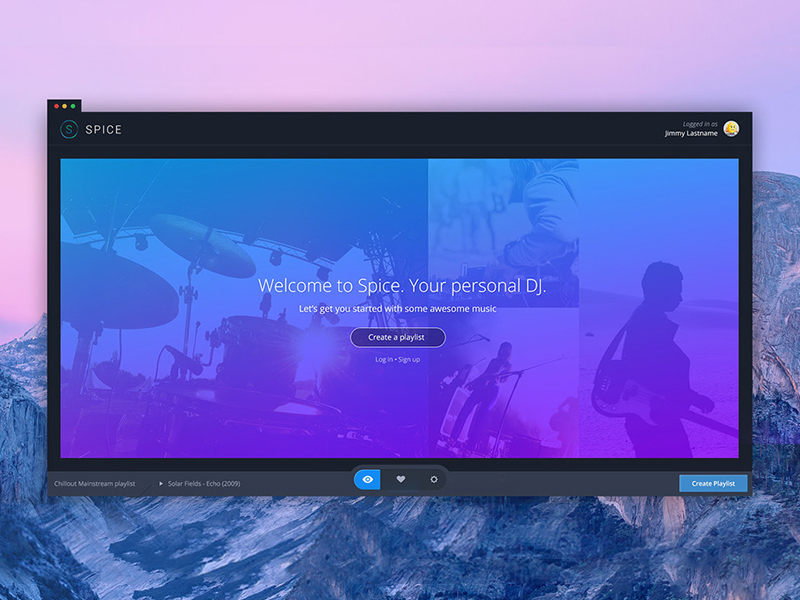The image in question is a digital screenshot approximately 20% wider than it is tall. At the center of the image, there is an Apple computer window, identifiable by the characteristic Apple menu options in the upper left corner, including the red, yellow, and green traffic light buttons. The background of this window is black.

In the upper left-hand corner of the window, there is a teal circle featuring a teal 'S' within it. To the right of this circle, written in all-white capital letters, is the word "SPICE". 

On the upper right side of the window, there is text indicating “Logged in as Jeremy [Last Name]”, adjacent to a profile picture of a yellow character.

The prominent feature of this image is a large banner occupying most of the display area. The banner features a gradient background transitioning from light blue at the top to purple at the bottom. The color scheme of the banner includes various shades of black and blue, and it contains different shots of a band as part of the design.

Overlaid on the banner in white text are the words "Welcome to Your Personal DJ" with a smaller text below that reads, "Let's get you started with some awesome music." Beneath this text is a dark blue button with the phrase "Create a Playlist" written in white.